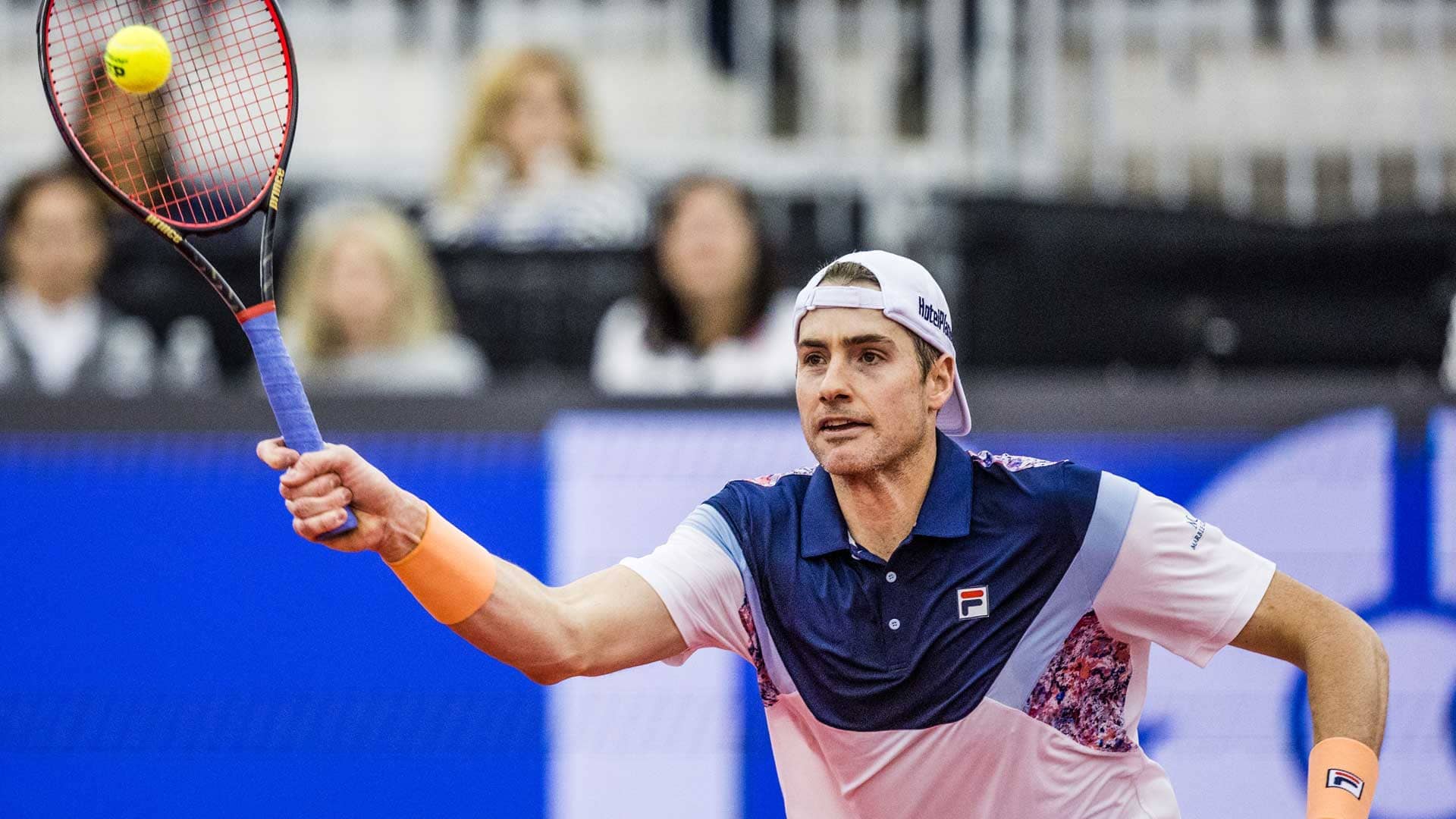In the foreground of the blurry image, a Caucasian man with a backwards white baseball cap, dark hair, dark eyebrows, stubble, and partially open mouth revealing his top row of teeth is captured mid-swing during a tennis match. His right arm, tensed with visible veins, is raised holding a blue-handled racket poised to strike a yellow tennis ball. He wears light orange Fila wristbands and a button-up polo shirt, which features a blue collar and placket with light blue and pinkish accents on the chest and sleeves, along with a Fila emblem. The action unfolds in front of a stadium fence lined with black and white seats, and the vague figures of spectators can be seen in the bleachers, though their faces are blurred. A partially visible blue and white sign is also present in the background.